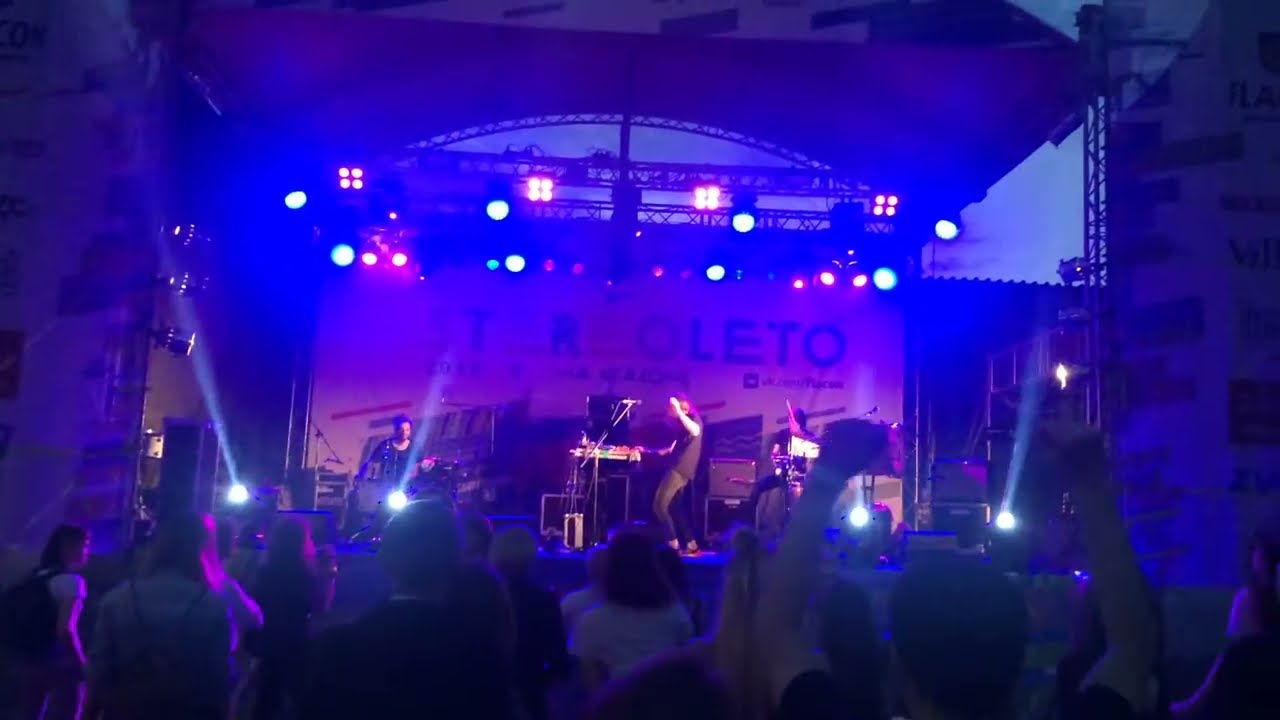The photograph captures an outdoor concert under a canopy with the blue sky visible in the background. The view is from the back of the audience, where several concertgoers, with their hands raised and some holding up cell phones, are engaged with the performance. The stage features a keyboardist at the center, flanked by a guitarist on the left and what appears to be a bass player on the right. There is also a drummer in the back, partially visible with his hand poised to strike a drum. The stage is illuminated by multiple lights, including four spotlights from the front that cast a blue hue over the scene. The backdrop displays a large banner with the partially obscured text "ST-REOLETO." The concert appears to be modest in size and has an intimate feel, suggesting a local or smaller-scale event.